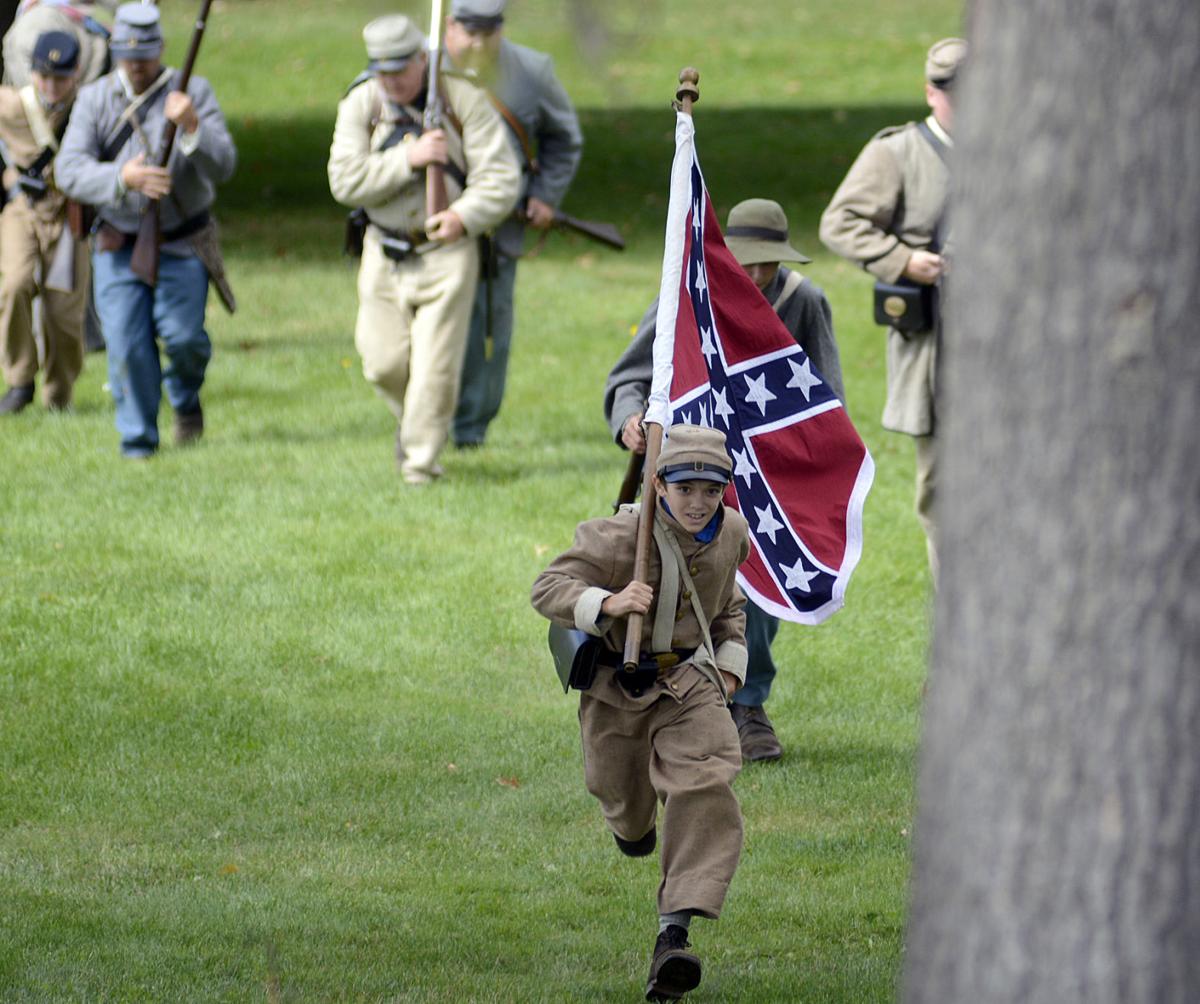This photograph captures a dynamic Civil War reenactment scene, where a group of people, dressed in historical uniforms, runs across a grassy field towards the camera. The participants wear a variety of uniforms, ranging in colors from navy blue to beige, brown, and gray, indicating both Union and Confederate soldiers. In the foreground, a young boy, approximately 8 to 11 years old, stands out in his tan-colored Civil War-era outfit. He is prominently holding a large Confederate flag on a wooden flagpole over his right shoulder. The image is focused on the advancing group, with older men in the back wielding flintlock-style rifles, slung over their shoulders. The scene is set against a somewhat blurry background, featuring a tree trunk in the upper right-hand corner, emphasizing the action and movement of the reenactment.